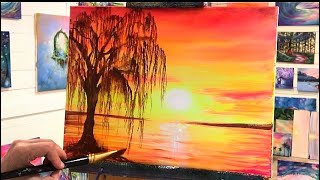In the foreground of the image, a brown hand with short nails delicately holds a black and gold-tipped paintbrush, poised to add details to a vibrant painting. The painting itself features an ethereal scene dominated by a drooping black weeping willow tree on the left, its branches cascading down towards a reflective body of water. The centerpiece of the painting is a radiant yellow sun, casting its glow amidst a dramatic sky painted in hues of red, orange, and yellow, which is mirrored on the surface of the water below. The beach at the base of the tree is depicted in deep black, adding contrast to the vivid colors of the sunset. Surrounding this focal painting are other canvases adorned with various scenes and colors, suggesting a gallery-like setting filled with the artist's diverse creations, though their specific details remain elusive in the background.